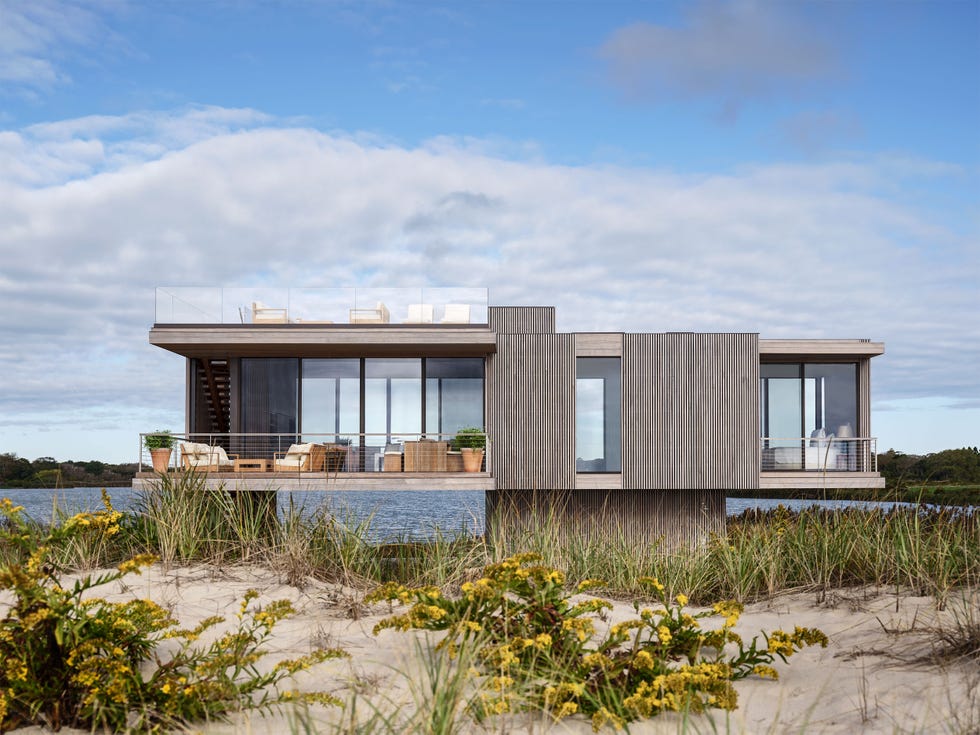The image depicts a modern, one-story, rectangular house with a flat roof and abundant windows, designed to appreciate the surrounding views. The house, which has gray trim, is elevated on concrete pillars or piers above a beachside setting with sand, plants, and some grass. In the foreground, there is a white sandy beach interspersed with green bushes featuring yellow flowers and patches of grass. To the left of the house, a deck furnished with lounge chairs, pots with plants, and a railing can be seen. This deck is connected by a set of stairs leading to the rooftop, where additional chairs are placed, enhancing the overall leisure space. The interior, partly visible through the numerous windows, reveals a bed positioned on the far right. The house overlooks a tranquil lake, with trees lining the distant shore. The background rises to a light blue sky, decorated with fluffy white clouds, completing the serene coastal scene.